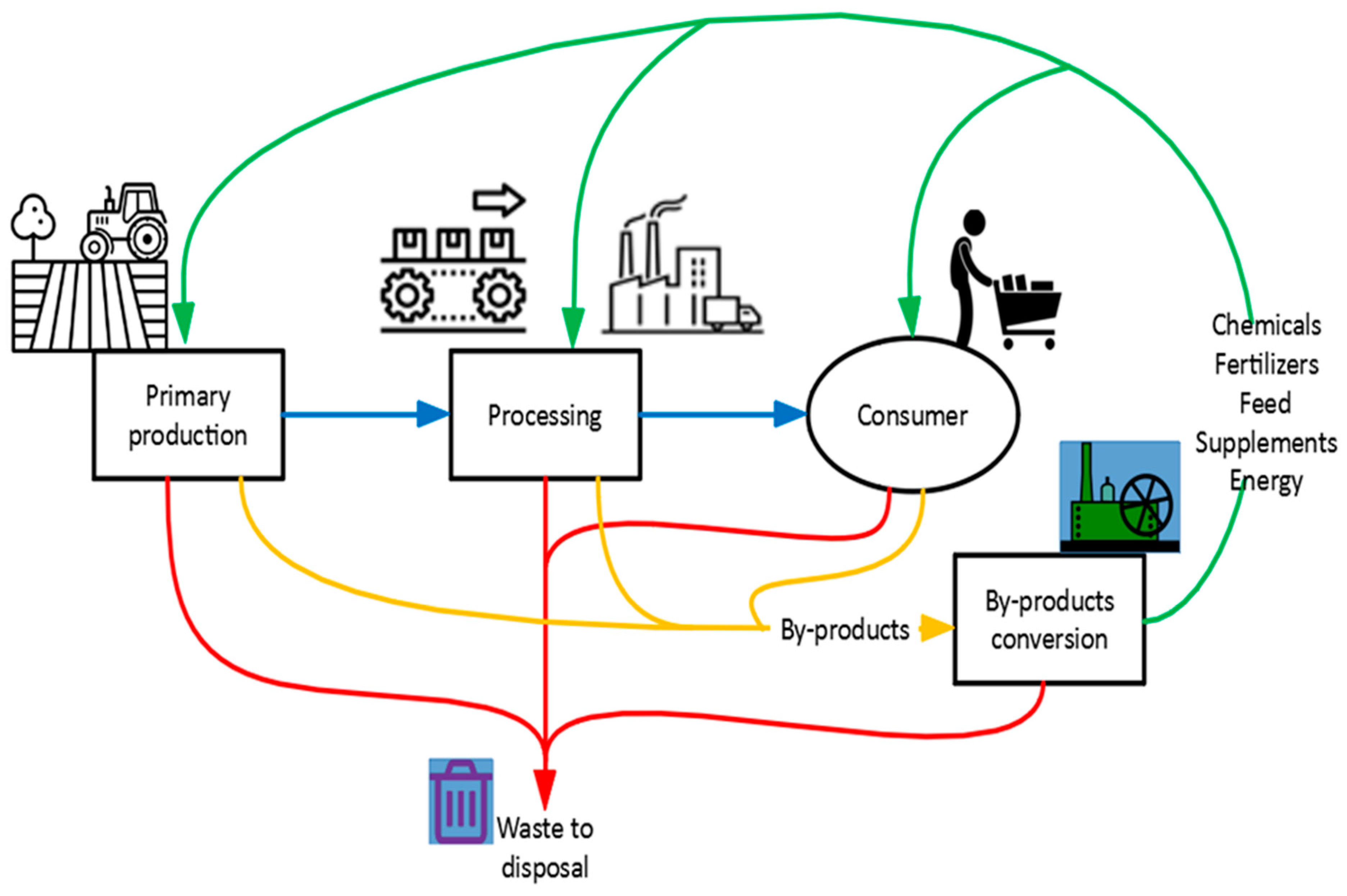The image is a detailed, computer-illustrated diagram depicting the flow of goods and resources from primary production to waste disposal. The color-coded flowchart uses green, blue, yellow, and red lines with arrows to signify various stages and connections in the production process. On the left side, a pictogram of a tractor illustrates primary production taking place on a field. This leads to the processing phase, represented by a factory building and cogs, signifying the transformation and packaging of goods. The diagram continues to the consumer stage, depicted by a stick figure pushing a grocery cart filled with groceries. It highlights how chemicals, fertilizers, feeds, supplements, and energy inputs are used throughout these stages, indicated by green arrows that intersect all phases. The final stage, waste disposal, is shown with a trash can icon, emphasizing the byproducts and packaging waste generated during the production and consumer phases. Text within the image labels each stage: primary production, processing, consumer, and waste disposal, providing a clear understanding of the cyclical nature of resource use and waste generation.